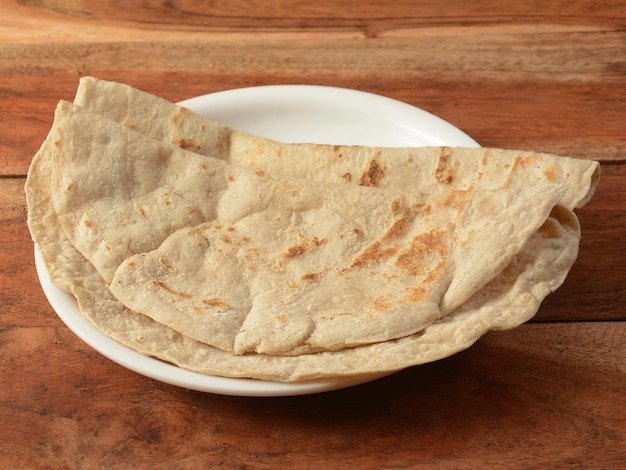A photograph captures a rustic, brown wooden table with visible grain and seams, resembling a picnic table. Centered on the table is a simple, white diner-type plate, slightly smaller than the two folded flatbreads it holds. The flatbreads, which could be naan or tortillas, are folded in half, taco-style, with one lying atop the other. Their tan surfaces are accented with golden-brown spots from recent toasting or grilling. The folds and overall arrangement suggest recent warming, adding a subtle tactile contrast to the image.